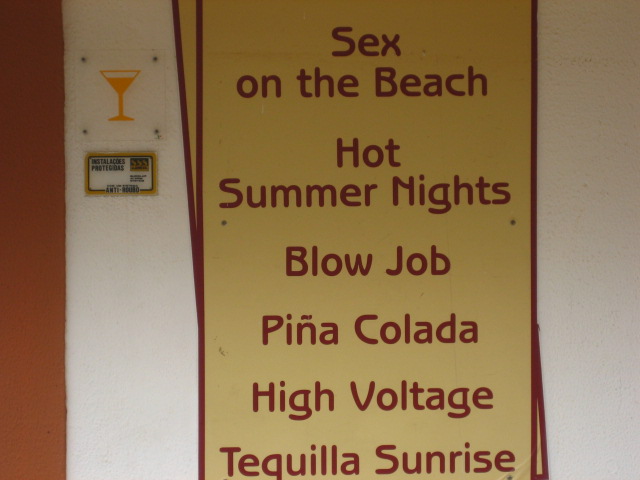This color photograph, in landscape orientation, features the cover of a cocktail menu poster designed with a striking aesthetic. The background is primarily white, showcasing two overlapping vertical segments that carry a yellow background with contrasting red lettering. In the top left corner, there is a gold martini glass icon, accompanied by an unreadable small black and white text box underneath it. The drink names are prominently displayed in red lettering arranged vertically from top to bottom. The list includes: Sex on the Beach, Hot Summer Nights, an intriguingly labeled Blowjob (which is flanked by two asterisks on either side), Piña Colada, High Voltage, and finally Tequila Sunrise at the bottom. The menu also has an elaborate design feature with a red outline that accentuates its visual appeal. The overall style is a realistic photographic representation of this prominently printed cocktail menu cover.